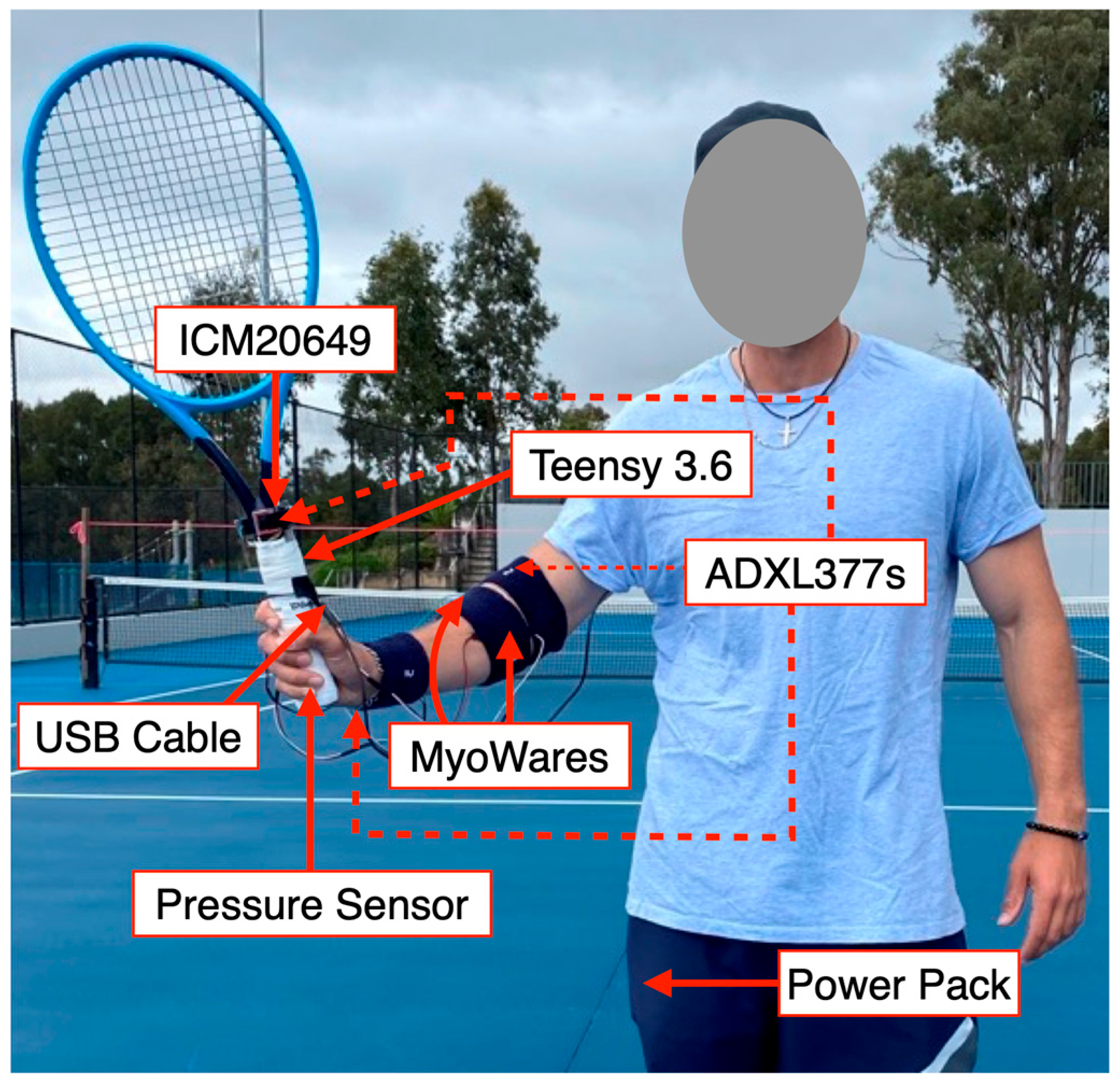The image depicts a man playing tennis on a green tennis court under cloudy skies, with lush green trees in the background. He is wearing a light blue t-shirt, darker blue pants, and a cross necklace. His face is obscured by a grey circle to maintain his anonymity. The man is holding a blue tennis racket with electronic attachments connected to his forearm and wrist via blue straps. Several labels, with red arrows and white rectangles featuring black text, point to various components of the setup. These include a Power Pack in his pocket, a Teensy 3.6 on the racket's handle, an ICM-20649 on the racket stem, an ADXL377S on his wrist, MyoWare's on the elbow brace, a USB cable running from the racket down his sleeve, and a pressure sensor on the racket's handle. The detailed labels suggest a sophisticated system for possibly monitoring or enhancing his tennis play.